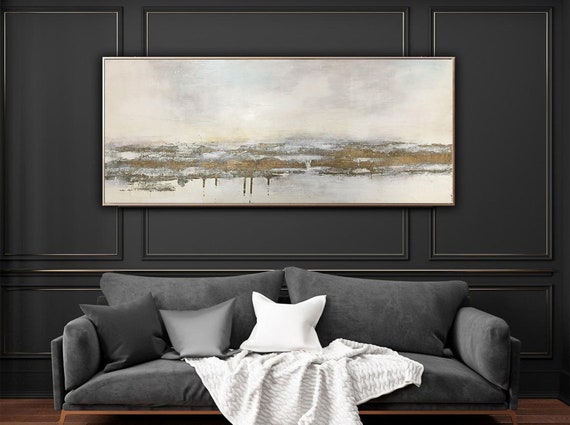This photograph captures an elegantly designed living room with dark charcoal gray walls adorned with intricate batten and picture frame molding. A striking horizontal abstract painting, approximately six to eight feet long, hangs above a modern gray sofa. The painting, which features a serene, gauzy scene with horizontal gold, silver, and blue lines, adds a touch of sophistication to the space. The sofa, which has two large gray cushions and wooden legs, is tastefully decorated with square throw pillows in dark gray, light gray, white, and silver hues, along with a white blanket casually draped over it. The room is accentuated by the rich brown hardwood flooring, creating a cohesive and inviting atmosphere. The photograph captures a direct, head-on view of the sofa and the wall, emphasizing the stylish artwork and contemporary furniture arrangement.